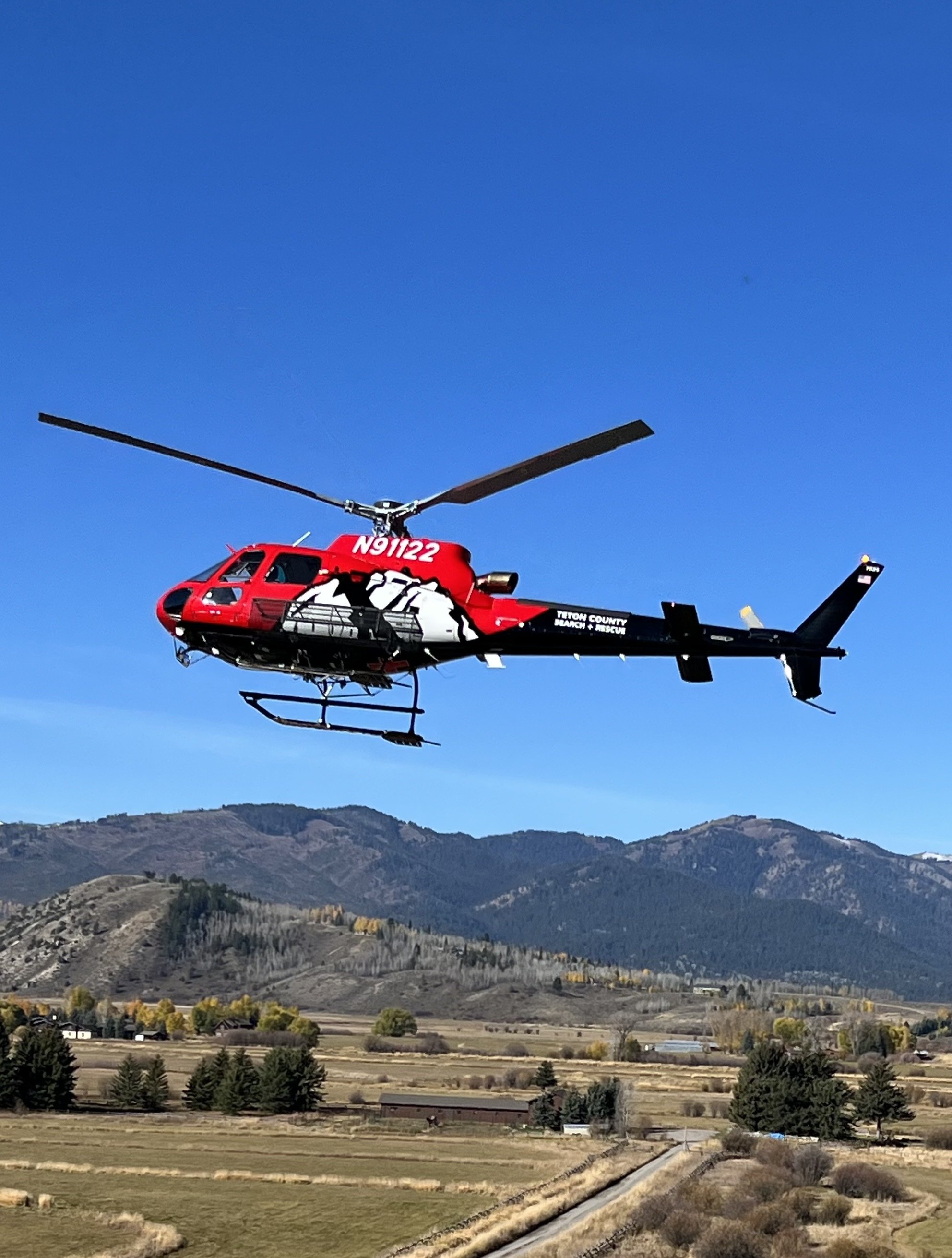In this outdoor photograph, the primary focus is a red helicopter with a white middle section and a black tail, marked with the ID number N91122. The helicopter appears stationary with its propeller blades still, and it is oriented towards the left of the image. The scene unfolds beneath a clear, light blue sky that occupies the top two-thirds of the photograph. Below, an aerial view captures a vast rural landscape featuring a gray asphalt road that stretches from the center bottom towards the top right corner. Adjacent to this road lies a rectangular brown building with a gray roof, situated in an area adorned with fields, small squat fences, tall yellow grasses, and scattered green trees. The horizon reveals mountain ranges covered in a mix of gray rock, green vegetation, and tall trees, with some peaks showing patches of snow. This serene yet detailed scene encompasses flat fields and rolling hills, extending into distant, lush mountains, all basking under the expansive sky.